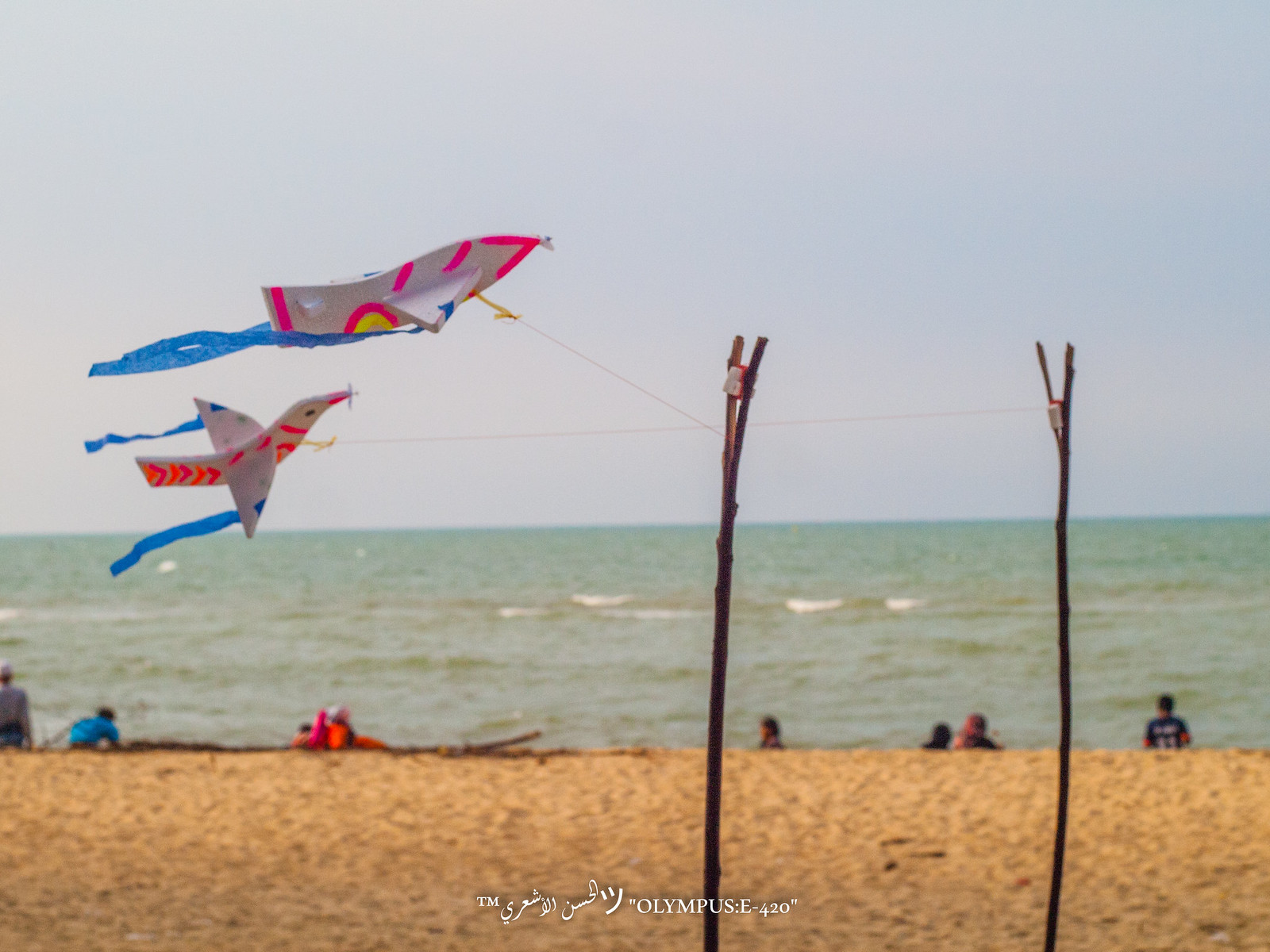This photograph captures a serene beach scene with a sandy foreground and a flat, somewhat choppy ocean in the distance. The sky overhead is overcast, casting a grayish hue over the landscape. Scattered along the shoreline are small groups of people, blurred and seemingly dressed warmly, suggesting it might be a chilly day. Prominently featured in the foreground are two forked sticks planted in the sand. Each stick has strings tethered to red, white, and blue kites—one resembling a bird, while the shape of the other is less distinct. These kites float freely in the breeze blowing from right to left. The photograph is signed with a trademark in Arabic writing, and the camera model "Olympus 420" is noted at the bottom.